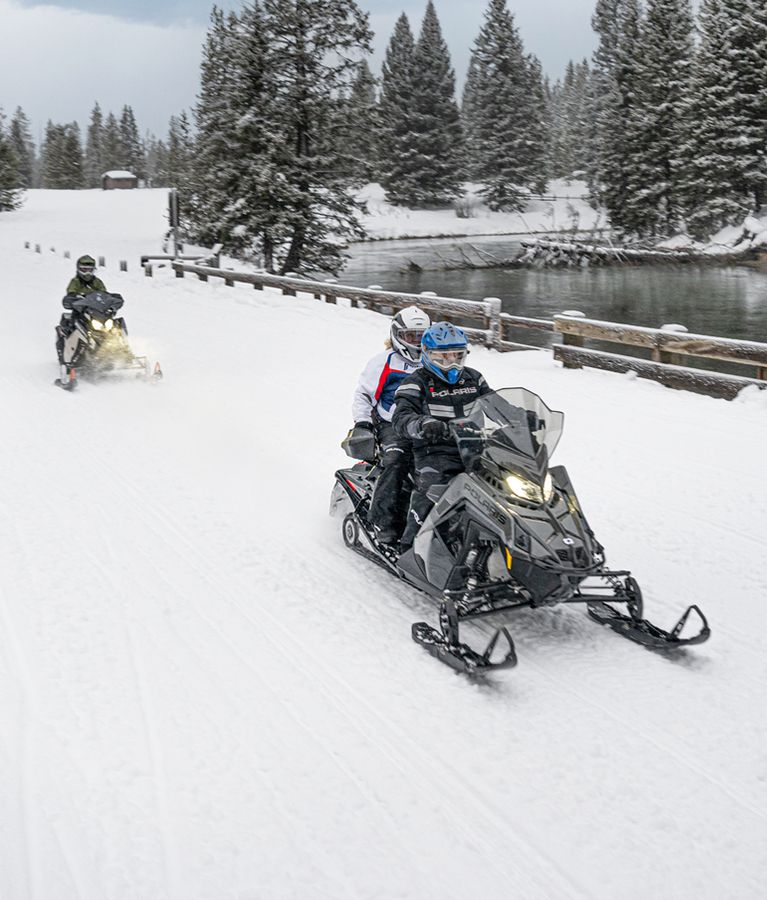In this winter scene, a snow-covered landscape features prominently, with a light gray sky and clouds adding to the chilly atmosphere. Snow-laden evergreens frame a distance view wherein a wooden fence separates the viewer from a body of water. A building is visible off in the distance.

In the foreground, two black snowmobiles are in motion, traversing a snowy path guarded by the wooden fence. The first snowmobile carries two people: the rider at the front is dressed in black with a light blue helmet, while the passenger wears a red, white, and blue jacket, dark pants, and a matching white and blue helmet. Both snowmobile headlights are on. The second snowmobile trails behind, ridden by a single individual clad in black. 

This dynamic photo captures the brisk outdoor activity during daylight hours, encapsulating the essence of a cold yet invigorating winter's day. Colors in the scene include striking contrasts of black, gray, blue, red, yellow, and dark green, contributing to the vivid portrayal of this winter adventure.